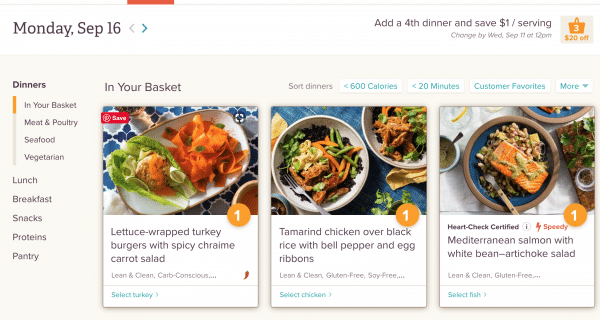This is a detailed screenshot of a menu planning app, with the current date set to Monday, September 16th. On the left side of the screen, there is a comprehensive menu categorized into different meal types. The primary categories include "Dinners," "Lunch," "Breakfast," "Snacks," "Proteins," and "Pantry." 

Under the "Dinners" category, sub-tabs are available for further navigation, labeled as "In Your Basket," "Meat & Poultry," "Seafood," and "Vegetarian." The central focus on the screen is the "In Your Basket" tab, which lists three items presumably added for purchase. 

The first item on the list is "Lettuce Wrapped Turkey Burgers with Spicy Prawn Carrot Salad." Following that is "Tamarind Chicken Over Black Rice with Bell Pepper and Egg Ribbons," and the third item is "Mediterranean Salmon with White Bean Artichoke Salad." 

At the top of the screen, there is an enticing offer displayed: "Add a 4th Dinner and save $1 per serving." This promotional message is likely aimed at encouraging users to add more items to their basket for additional savings.